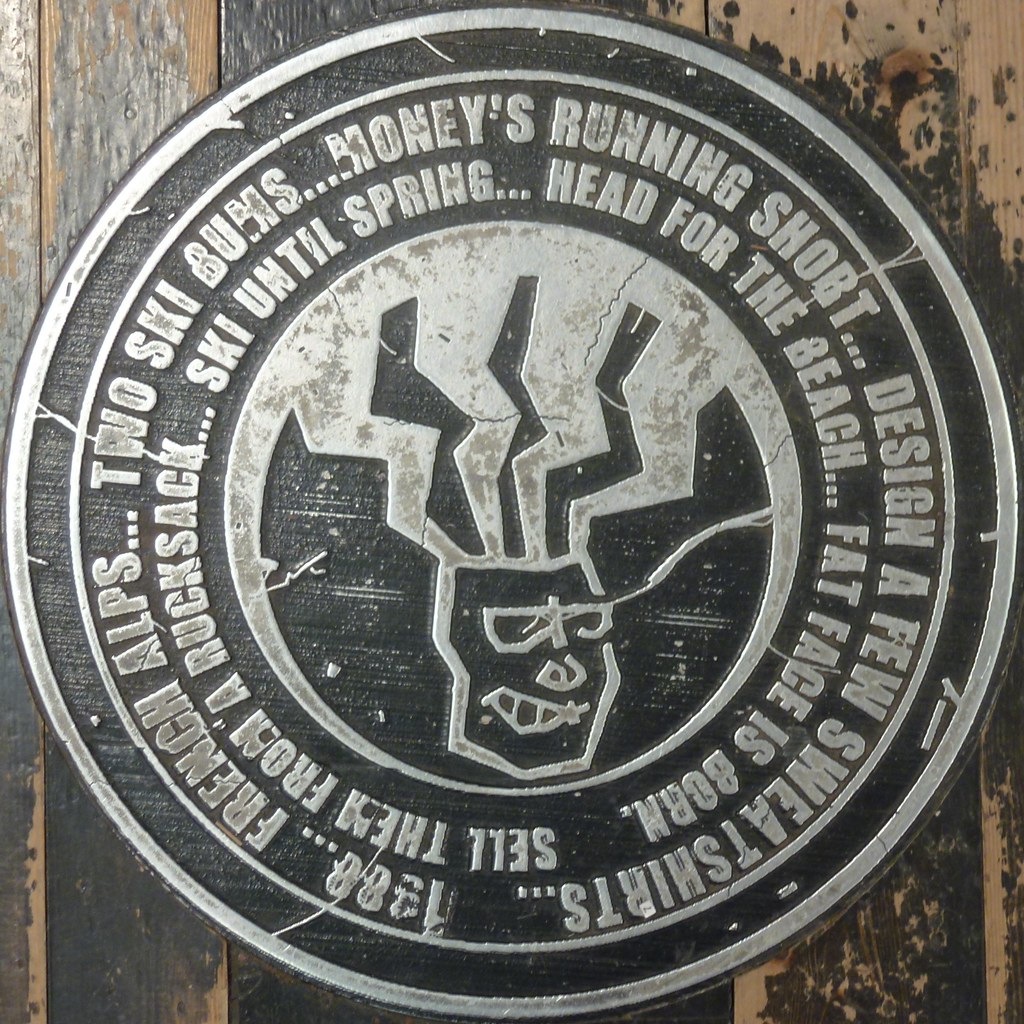The photograph captures a large, round metal plaque embedded in a brownish wooden wall streaked with black. The plaque resembles a manhole cover but with a decorative design, featuring worn, raised silver areas and recessed black sections. Inscribed around the outer circle of the plaque is the text: "1988, French Alps, two ski bums, money's running short, design a few sweatshirts, sell them from a rucksack, ski until spring, head for the beach, fat face is born." At the center of the plaque is a grinning face with wiry, electric shock-like hair, adorned with what appear to be goggles or sunglasses. The overall appearance suggests that the plaque has been walked over or touched frequently, adding to its worn charm.